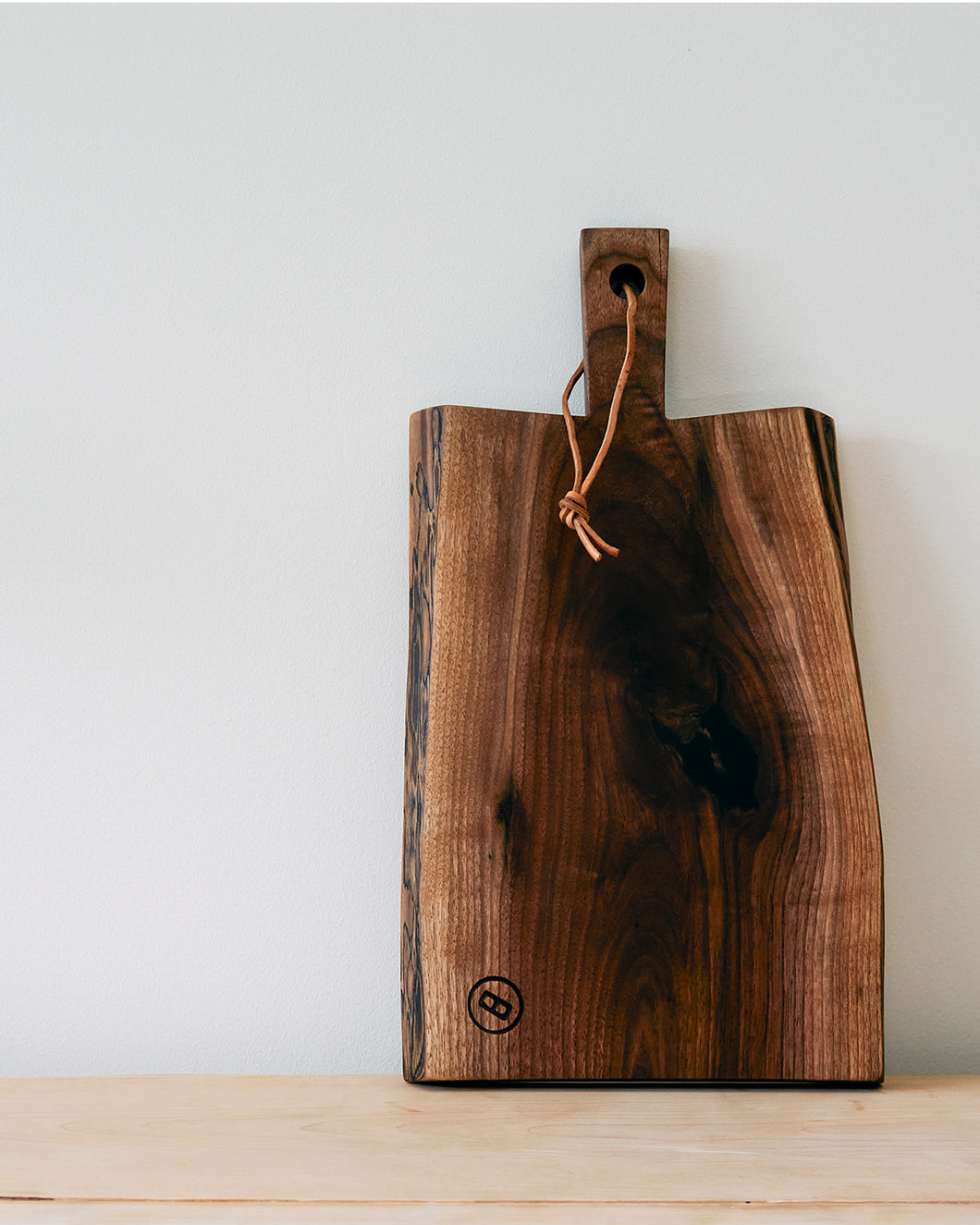This photograph features an elegant and robust cutting board, notably crafted from a thick, dark wood, possibly walnut. Positioned upright, the board leans against a stark white wall and rests on a light wooden table with a raw, unpainted finish. The cutting board itself is rectangular with live, uneven edges which accentuate its natural aesthetic. 

Its handle is distinctively fashioned from the same dark wood, featuring a hole through which a leather cord is threaded and knotted, enabling easy hanging. The wood grain is prominently visible across the entire board, adding rich texture and visual depth. In the bottom left corner of the board, there is a meticulously engraved emblem depicting a bee or possibly the letter 'B' within a circle. The elaborate engraving further enhances the board’s rustic charm. 

Overall, the setting and the intricate details of the wood are captured with clarity, offering a comprehensive view of the board's craftsmanship and natural beauty.